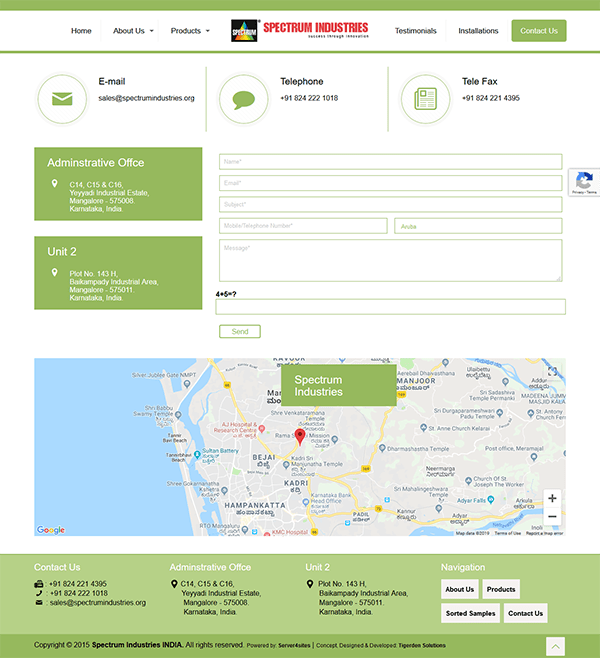This image is a screenshot of the Spectrum Industries website. The top navigation bar features "Spectrum Industries" prominently in red font in the center. On the left side of the bar, there are menu options including a "Home" button, and "About Us" and "Products" sections, each accompanied by a drop-down arrow. The company logo, which is a yellow, red, and light green triangle inside a black square, is also visible.

To the right of "Spectrum Industries" are additional menu options for "Testimonials" and "Installations." A solid green "Contact Us" button is positioned to the far right.

Below this bar, the contact email "sales@SpectrumIndustries.org" is displayed. Directly beneath the email, the phrase "Administrative Office" appears, followed by the company's address which includes "Unit Two." At the bottom of the page, a map is shown.